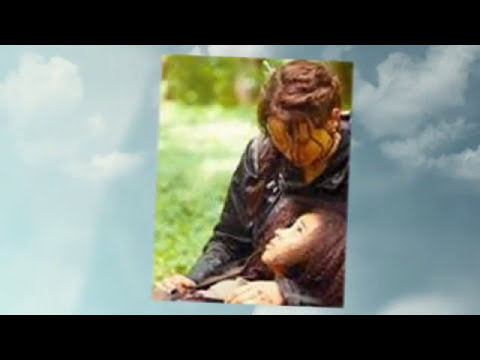The photograph, framed by black bars at the top and bottom, captures a poignant moment against a backdrop of a bluish-gray sky dotted with off-white clouds and sunbeams streaming from the left. Central to the image are two females, both with brown hair; the older woman has her hair in a long braid and wears a black leather jacket, while the younger girl, characterized by her tight curls, looks up at her with a plaintive expression. The older woman, a white female dressed in a dark blouse, gazes down at the girl with closed eyes, her face conveying a comforting assurance amidst a shared sadness. The green grass and indistinct foliage in the background add an organic, serene touch to the intimate, unposed scene.